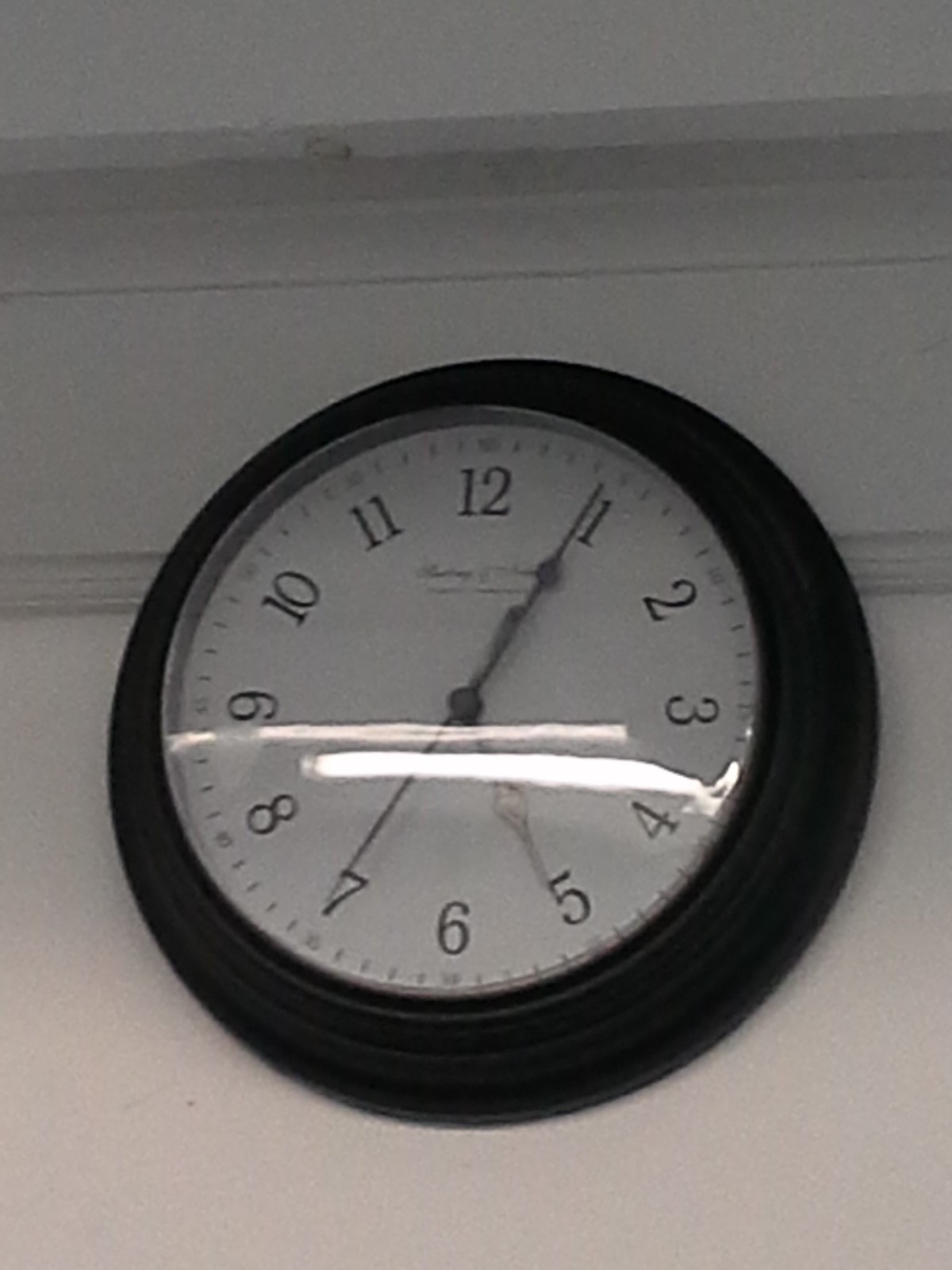In this somewhat grainy black and white photograph, the background features a monochromatic wall with a distinguished piece of crown molding running horizontally along the top. Positioned against this wall is a round clock with a black exterior frame and a white clock face. The clock displays the time as 5:04, with the second hand aligned near the 7. Below the clock, the wall appears brighter, almost a stark white, gradually transitioning to a much darker, almost gray shade as your gaze moves upward towards the top of the image.